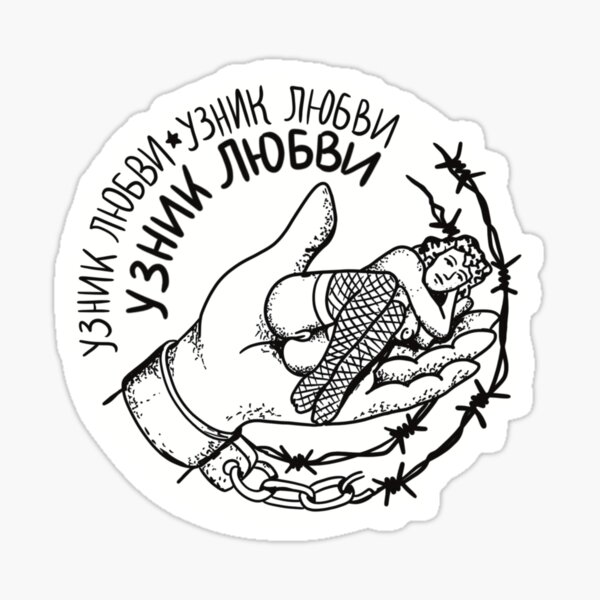The image depicts a circular emblem presented in black and white. The emblem features a left hand, palm open, with a chain attached to the wrist that connects to a section of barbed wire encircling the edge of the circle. In the center of the palm rests a partially nude woman dressed in fishnet stockings. The design includes text in a foreign language using the English alphabet in all capital letters. The overall theme appears to hint at a serious issue such as sex trafficking or imprisonment. The emblem’s rough, imperfect circular design, the barbed wire, and the chained hand collectively suggest a theme of captivity and control.